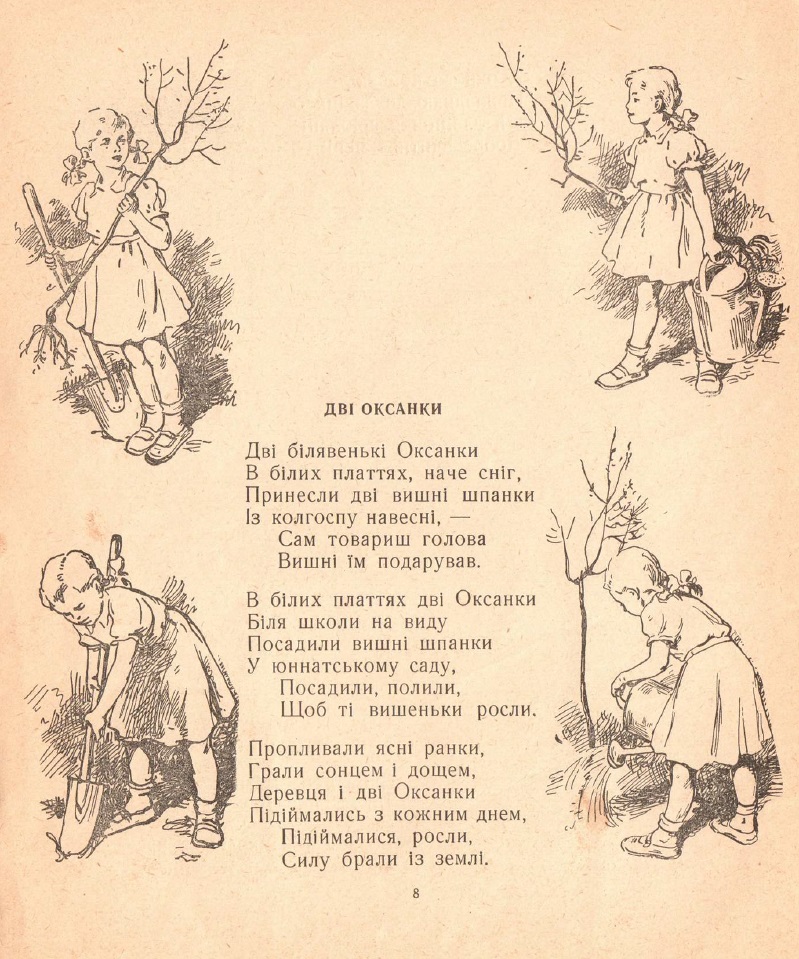This image resembles a vintage children's storybook page, rendered on aged, yellowed paper reminiscent of a tea-stained color. The central feature is a passage of text in bold, likely Russian, suggesting it may be a poem or story. Four pencil-drawn illustrations of a young girl with pigtails, clad in a 1940s-style dress, frame the text: one in each corner of the vertical rectangular page. In the top left, she is depicted with a shovel in her right hand and a tree sapling in her left. The top right shows her holding the sapling and a watering can. In the bottom left, she is seen diligently digging a hole with the shovel, while the bottom right captures her watering the newly planted sapling. The scene, rendered in shades of beige, black, and gray, evokes an old-fashioned, charming children's book illustration, with a focus on the sequence of planting and nurturing a tree.